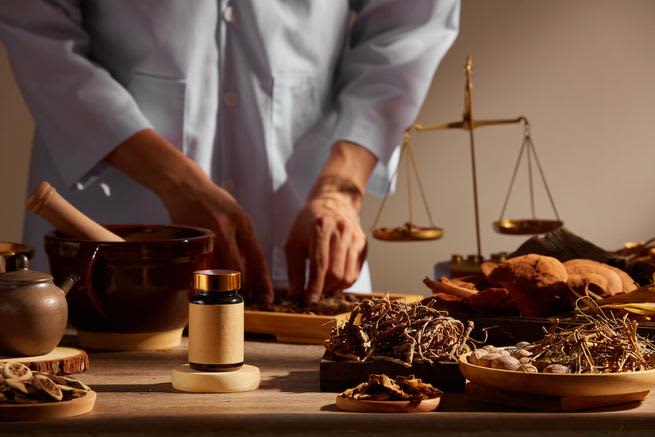The photograph focuses on a wooden table laden with various culinary tools and ingredients. In the foreground, there is a tannish, cream-colored bottle with a gold top, surrounded by wooden bowls and plates that contain what appears to be herbs, grass, or roots. A large bowl with a wooden pestle laid across it is also present. Among the items on the table are jars of seasoning and pots, along with a sandwich already prepared on the lower left side. Dominating the scene is a Caucasian man, presumably a chef, who is primarily visible from the chest down, dressed in a white coat and a blue shirt. His hands are actively engaged in preparing ingredients on a wooden plate. In the upper right quadrant of the image, there is a gold scale with two weights. The background is slightly blurred, and the setting appears to be a studio shot with a brown backdrop.